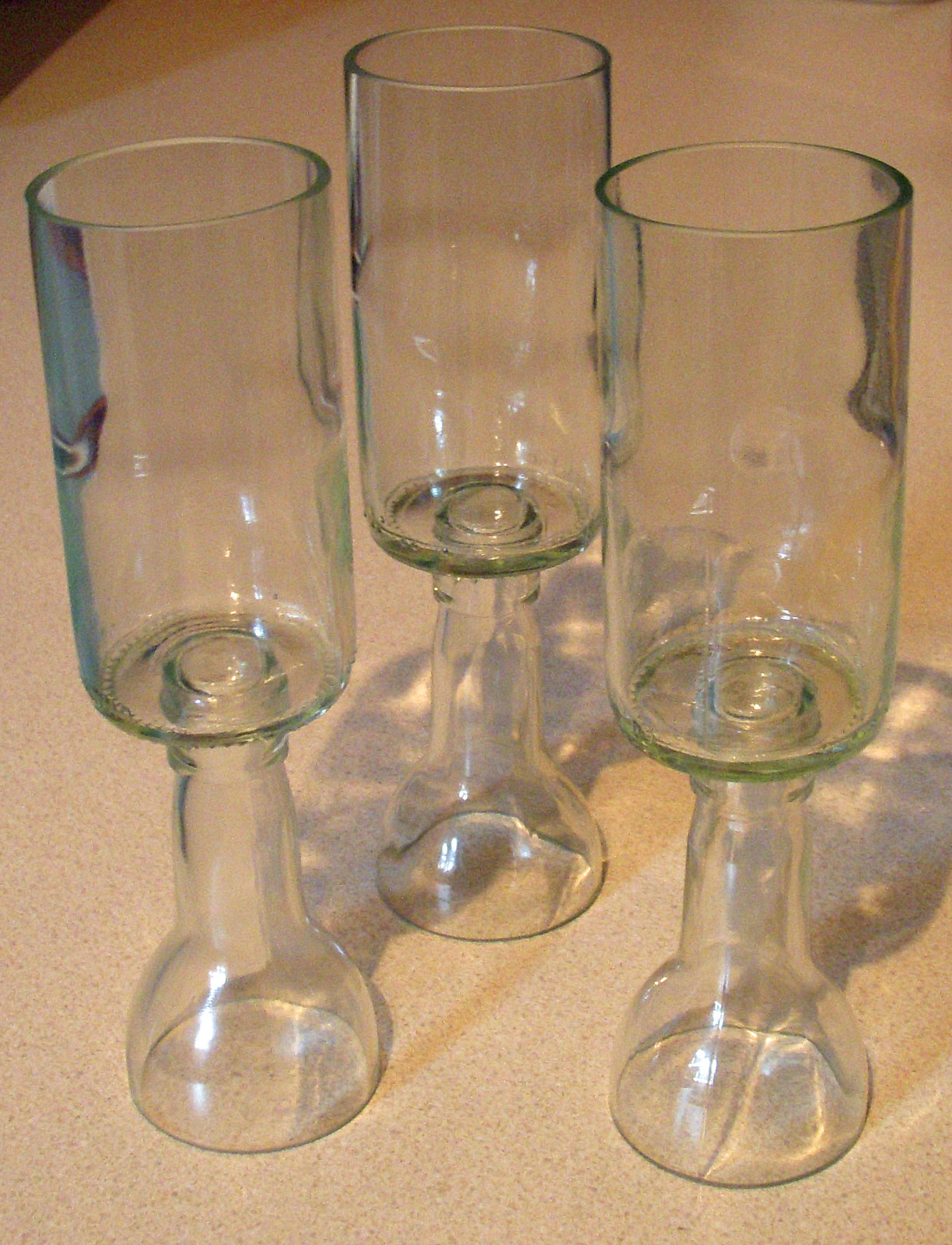This photograph features a trio of unusual, clear stemmed glasses arranged in a pyramid formation on an off-white, beige countertop with subtle gray speckles. The glasses, resembling modified wine glasses or potentially even candlestick holders, have cylindrical tops that give way to distinctive, thick, bell-shaped stems that flare out at the base, creating a bubble-like appearance. They are positioned with one glass in the center and the other two slightly lower on either side. The lighting in the scene is dim, with soft reflections casting dark gray shadows on the countertop behind the glasses, adding an intriguing play of light and shadow to the composition.